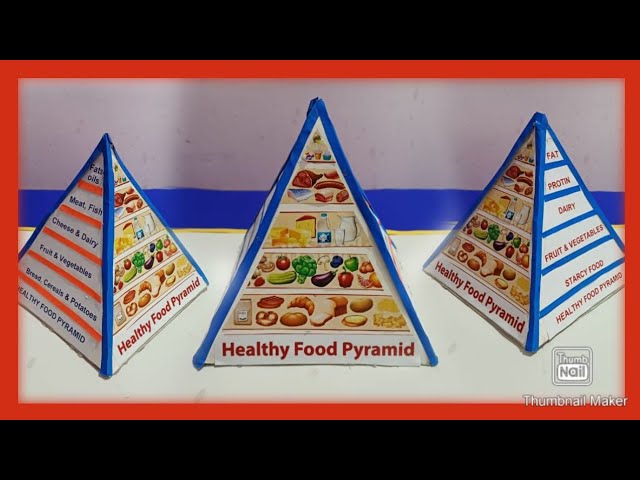The image is a relatively rectangular screenshot depicting a 5th grade class project centered around the Healthy Food Pyramid concept. The image is framed in black borders on the top and bottom, with a red rectangle inside those borders. Enclosed within this red rectangle is a display of three distinct food pyramids, each constructed by cutting and assembling printed triangular sections that illustrate the Healthy Food Pyramid. These triangles are taped together with painter's tape, forming three actual pyramid shapes that are placed on what appears to be a white table. The pyramids are outlined in bright blue and twisted in different directions.

The background is a blended gradient of bluish and pinkish hues, accompanied by a big blue stripe. Text reading "Thumbnail Maker" is visible in the bottom right corner. Each pyramid follows the same format: the base is labeled with starchy foods, followed by layers of fruits and vegetables, dairy, and protein, with a narrow top section for fats. Representative pictures of various foods are included within each segment, illustrating the recommended portions for a balanced diet according to the Healthy Food Pyramid guidelines.